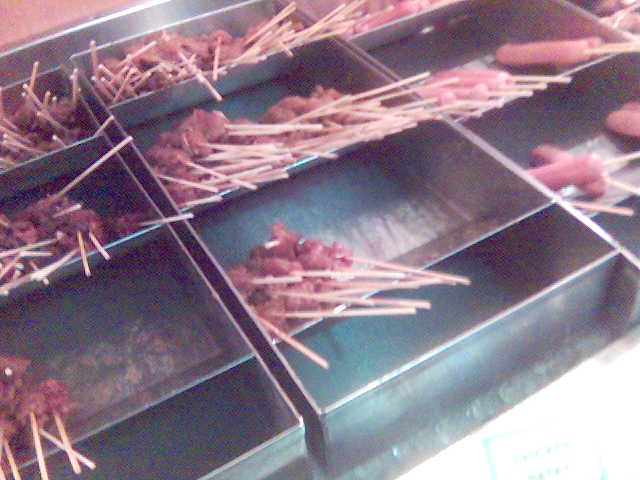The image depicts a set of metal trays arranged in a diagonal layout, likely in a commercial kitchen or restaurant setting. There are fourteen slots within these trays, of which twelve are occupied. Most trays hold wooden skewers, resembling small chopsticks or pine sticks, laden with bite-sized cubes of meat, appearing like beef or lamb with a reddish tint. Some skewers have small chunks that look breaded and golden, akin to chicken nuggets. Additionally, a few trays on the right contain skewers inserted into shiny sausages or hot dogs. The trays appear to have angled slots, possibly for draining or drying. The viewpoint is diagonal, capturing the trays from a side angle, with some glimpses of the surrounding area.